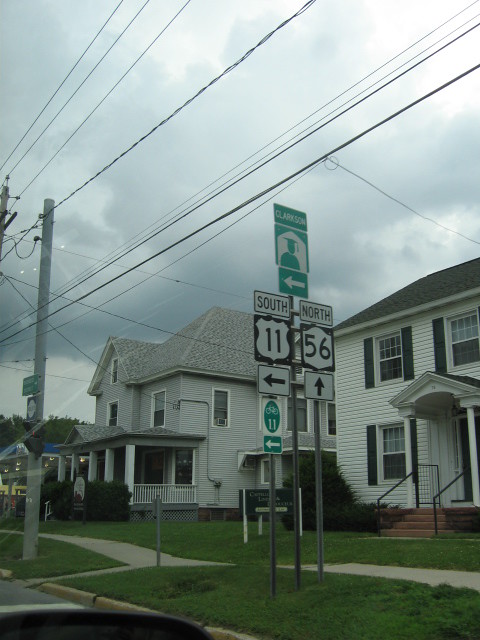The photograph portrays a neighborhood scene under an overcast sky with thick white clouds. It captures two prominent two-story homes. The home on the left is gray with a matching gray roof, accented by white posts and rails forming a front porch. To the right stands a white house with green shutters, a gray roof, and a brick staircase adorned with a black railing leading to the front door. Between a well-manicured green lawn and the street runs a sidewalk, flanked by several street signs. One silver post holds a sign showing 'South 11' with an arrow pointing left and 'North 56' with an arrow pointing up, while another silver post to the right bears a green sign with an image of a graduate and the word 'Clarkson' also pointing left. A yellow curb is visible at the bottom left corner of the photograph, as well as power lines stretching across the cloudy sky. The image appears to be taken from inside a car, with a part of the street visible in the foreground.